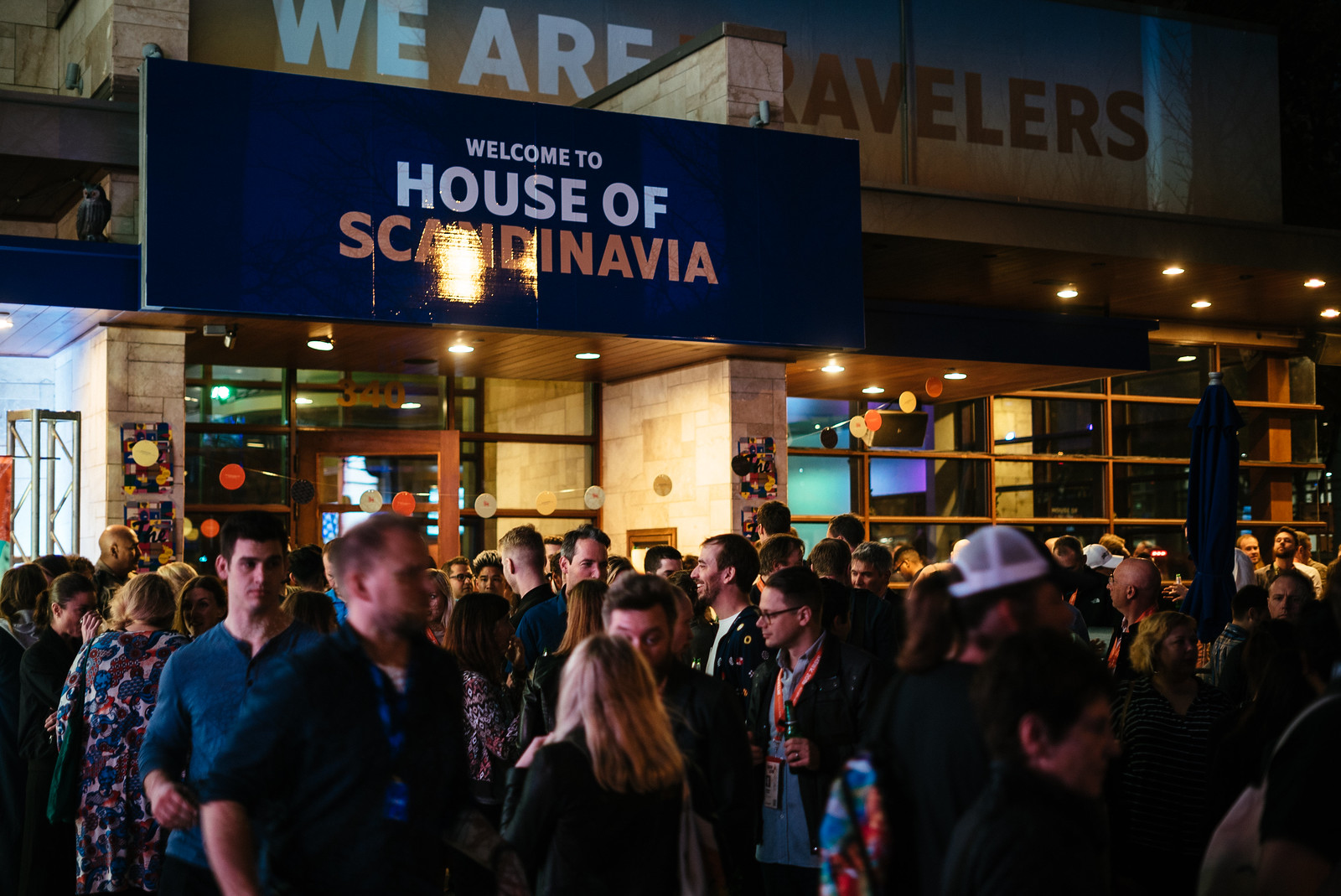In this night-time photograph, a diverse crowd congregates around the entrance of a building adorned with a prominent blue sign that reads, "Welcome to House of Scandinavia" in white and gold letters. The building itself stands out with a warm, golden hue, illuminated by lights above the entrance and the sign itself, providing the primary source of light in the otherwise dark scene. Above the main sign, additional text emblazoned on the building reads, "We are Travelers," with "We are" in white and "Travelers" in brown letters. The crowd, consisting predominantly of people in their 30s and 40s, features various individuals, including a man sporting a baseball hat and a ponytail. Some people appear to be entering the building while others are walking away, contributing to a lively, bustling atmosphere. The well-lit entrance and the activity around it suggest that this location could be a popular bar or nightlife venue.